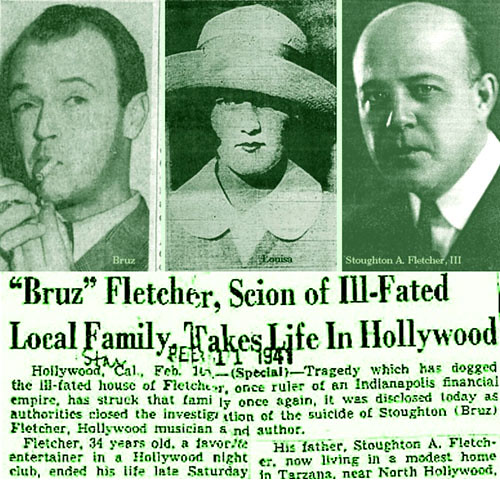The image is a black-and-white newspaper clipping, dating from February 11, 1941, as indicated by a faint stamp between the headline and the article. The clipping appears to be old-fashioned and is partially cut off at the bottom. At the top of the clipping are three vertically-aligned, portrait photographs of individuals: on the left is a man named Bruce, identifiable by his short hair and cigarette, with his hands up near his face; in the middle is a woman wearing a white-brimmed, old-fashioned hat and a thick-collared garment; and on the right is a severe-looking bald man in a suit. The headline reads, "Bruce (Bruz) Fletcher, scion of ill-fated local family, takes life in Hollywood." Below the headline, the article is arranged in two columns, starting with a few paragraphs before being cut off. This tragic news originates from Hollywood, California, and details the events surrounding Bruce Fletcher's life and demise.